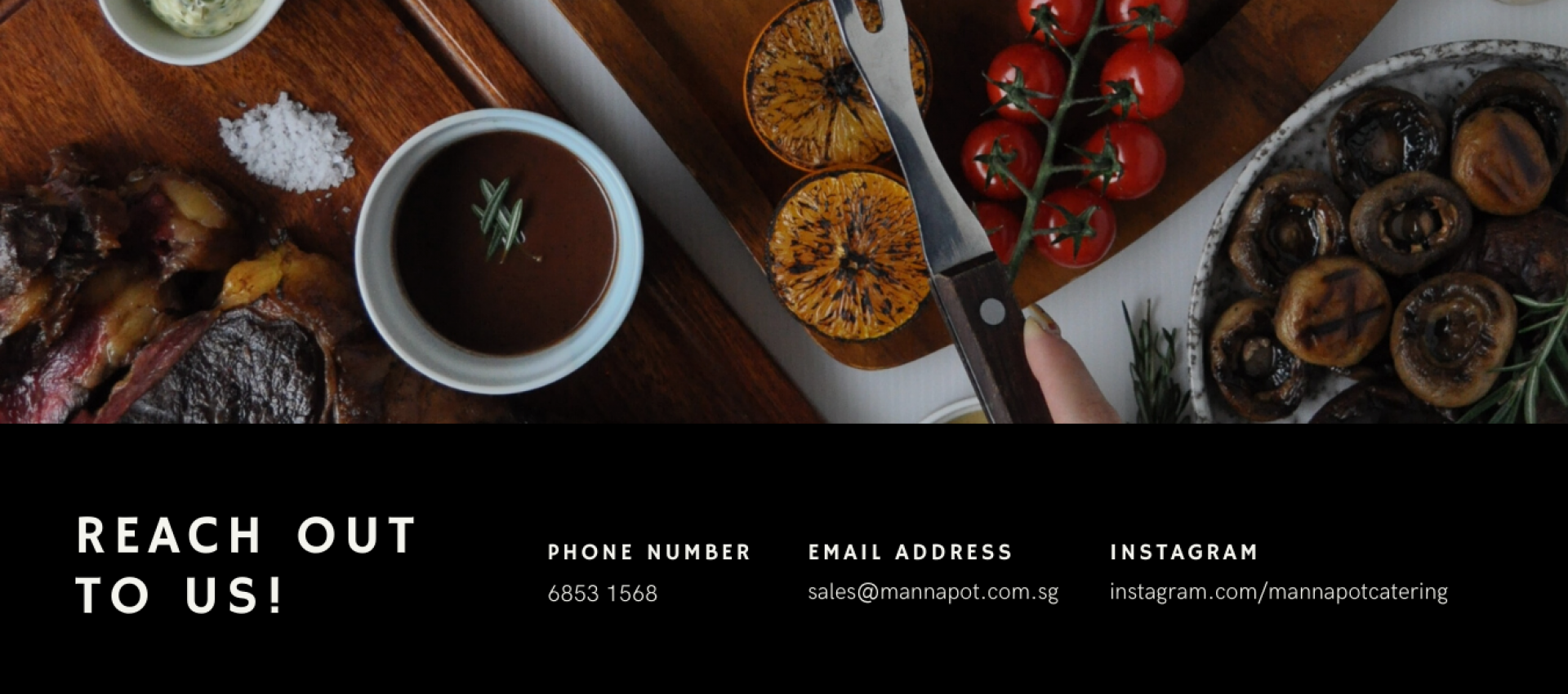In this visually compelling webpage image, the bottom half predominantly features a sleek black background. Anchored in the bottom left corner is the bold and inviting phrase "Reach Out to Us!" followed by a sequence of contact details. These include a phone number, an email address, and an Instagram link, all aligned horizontally to the right of the call-to-action text. Beneath these, smaller text provides further information, with all text displayed in white for stark contrast against the dark background.

The top half of the image commands attention with a vibrant and meticulously arranged food design. On the left side, there is a tempting display of sliced meat with a small white bowl containing brown sauce, possibly garnished with white seasoning or a scatter of white rice, all placed on a rustic brown table. Adjacent to this tableau, moving rightward, is a utensil with a polished brown handle, accompanied by a single finger visible, delicately holding the handle. Flanking the utensil are two slices of fruit and some ripe tomatoes, adding a pop of color to the scene. The far right section of this culinary display features a bowl filled with a scrumptious variety of food, resting on a light gray countertop. The entire arrangement is viewed from an overhead perspective, providing a comprehensive and aesthetically pleasing view of the delicious spread. This meticulous styling defines the top half, completing the vivid and engaging layout of the webpage.